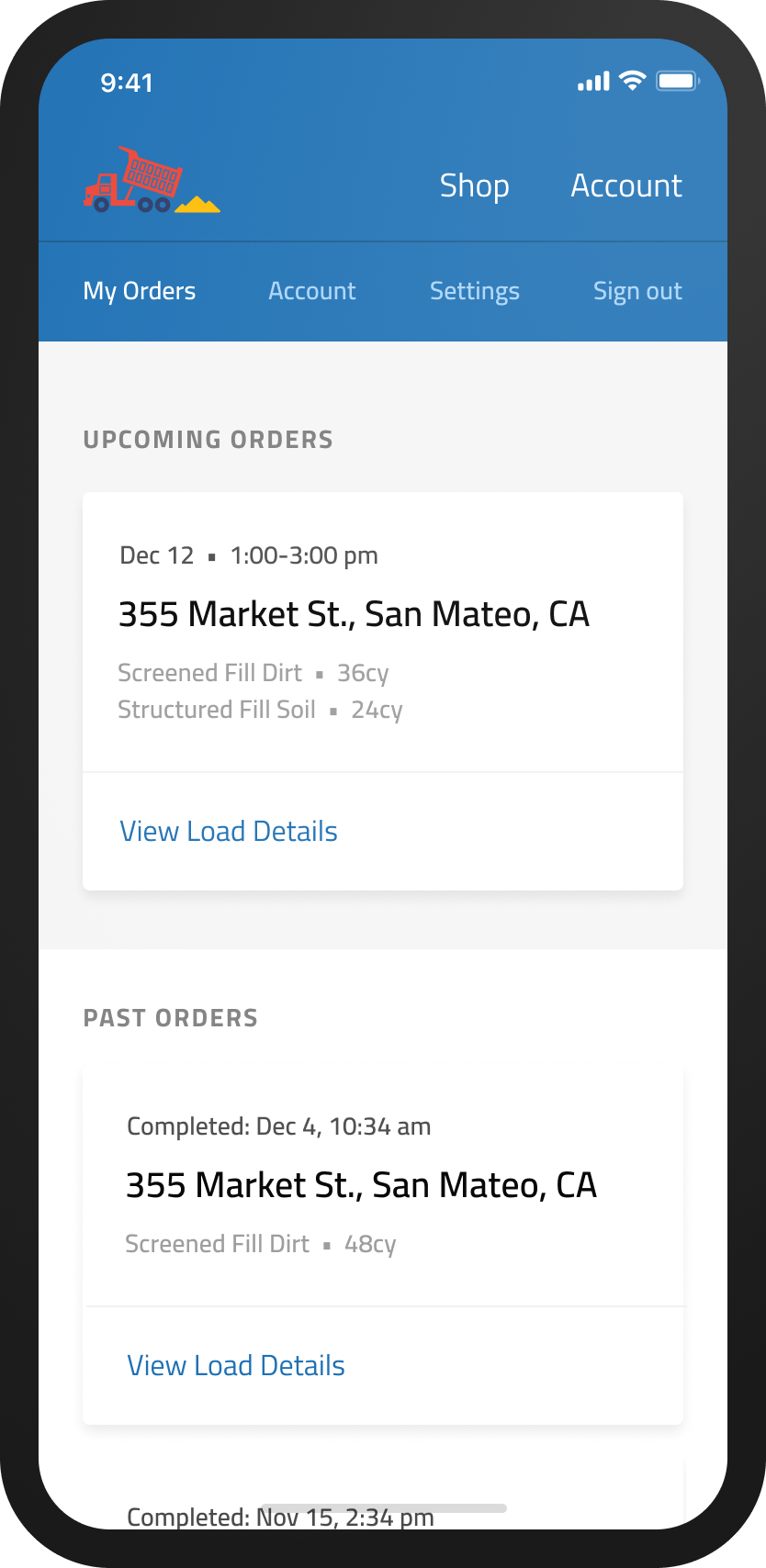Screenshot of a mobile application screen with a timestamp of 9:41 displayed on the top left. The top right corner shows full Wi-Fi signal strength and 100% battery charge. The header features a blue border with a red tow truck, depicted as a dump truck offloading what appears to be golden sand. Adjacent to this image, there are two buttons labeled "Shop" and "Account."

Beneath the header, there are four navigation tabs: "My Orders," which is currently selected, "Shop," "Account," and "Settings," followed by a "Sign Out" option. 

The main page showcases the section "Upcoming Orders," highlighting an order scheduled for December 12th between 1 PM and 3 PM at 355 Market Street, San Mateo, California. Below this, a clickable blue text that reads "View Load Details" is present.

Further down, a section for "Past Orders" is shown. It lists a completed order on December 4th at 10:34 AM at the same address, followed by another clickable "View Load Details" link. Another past order is partially visible, indicating completion on November 15th at 2:34 PM, but the details are cut off and not fully readable.